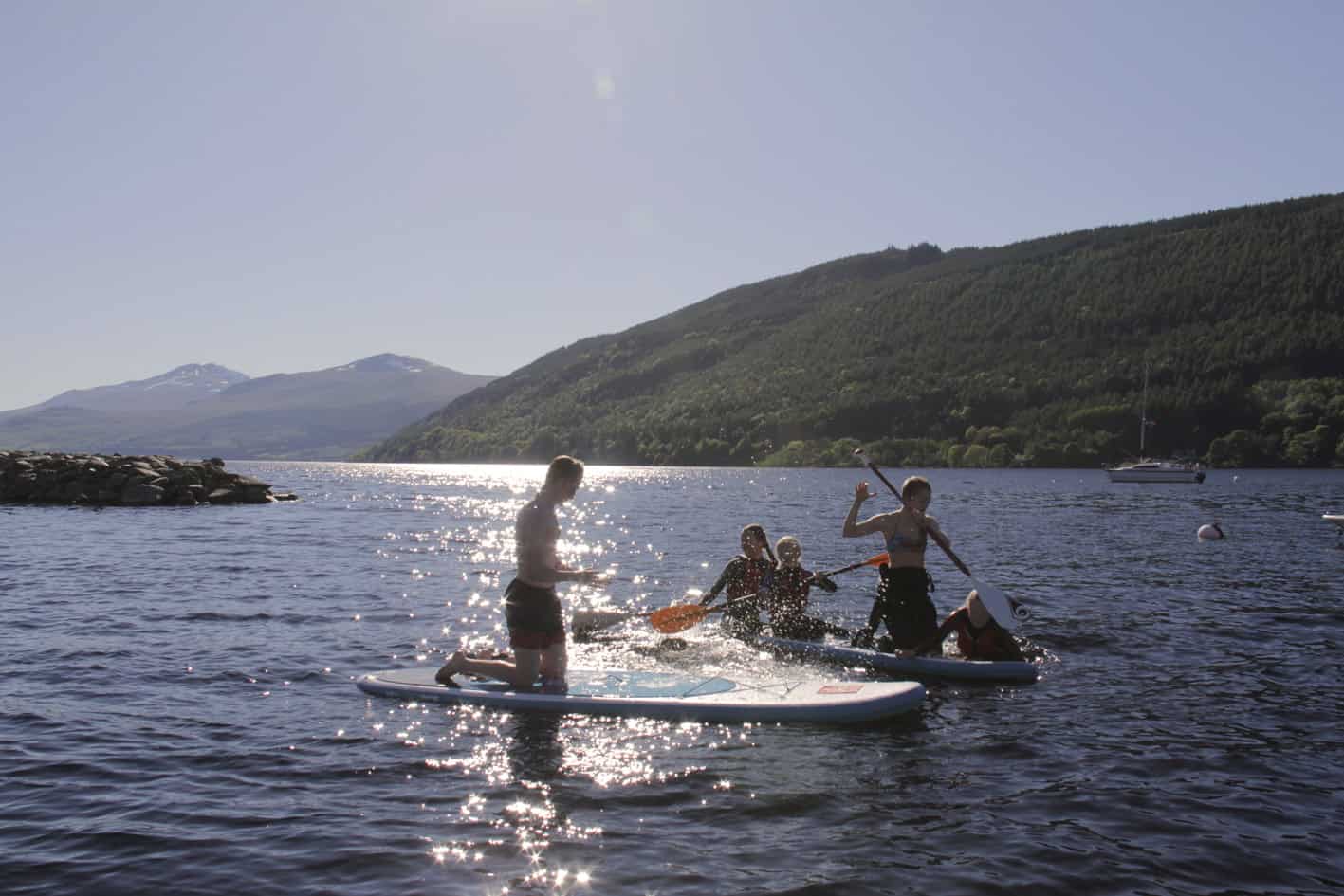On a warm and sunny summer day, a family enjoys a scenic outing on a tranquil lake surrounded by rolling, tree-covered hills and distant grayish mountains. The sky is a soft light blue, reflecting brilliantly off the water, which sparkles under the sun’s strong rays. In the foreground, a man in black swim shorts kneels on what appears to be a paddleboard or kayak, gazing at his family in the adjacent vessel. This family boat, likely a kayak or canoe, contains four visible members: a woman kneels in the front, and behind her sits two girls, with one of them distinguishable by her braided hair, and possibly a boy with them. The family uses long-handled oars to smoothly propel their craft. Along the shoreline, to the left, a small outcropping of rocks adds to the picturesque scene, along with a sailboat anchored to the right. The serene environment is accentuated by the gentle waves and the serene sparkle of the lake's darker blue waters.